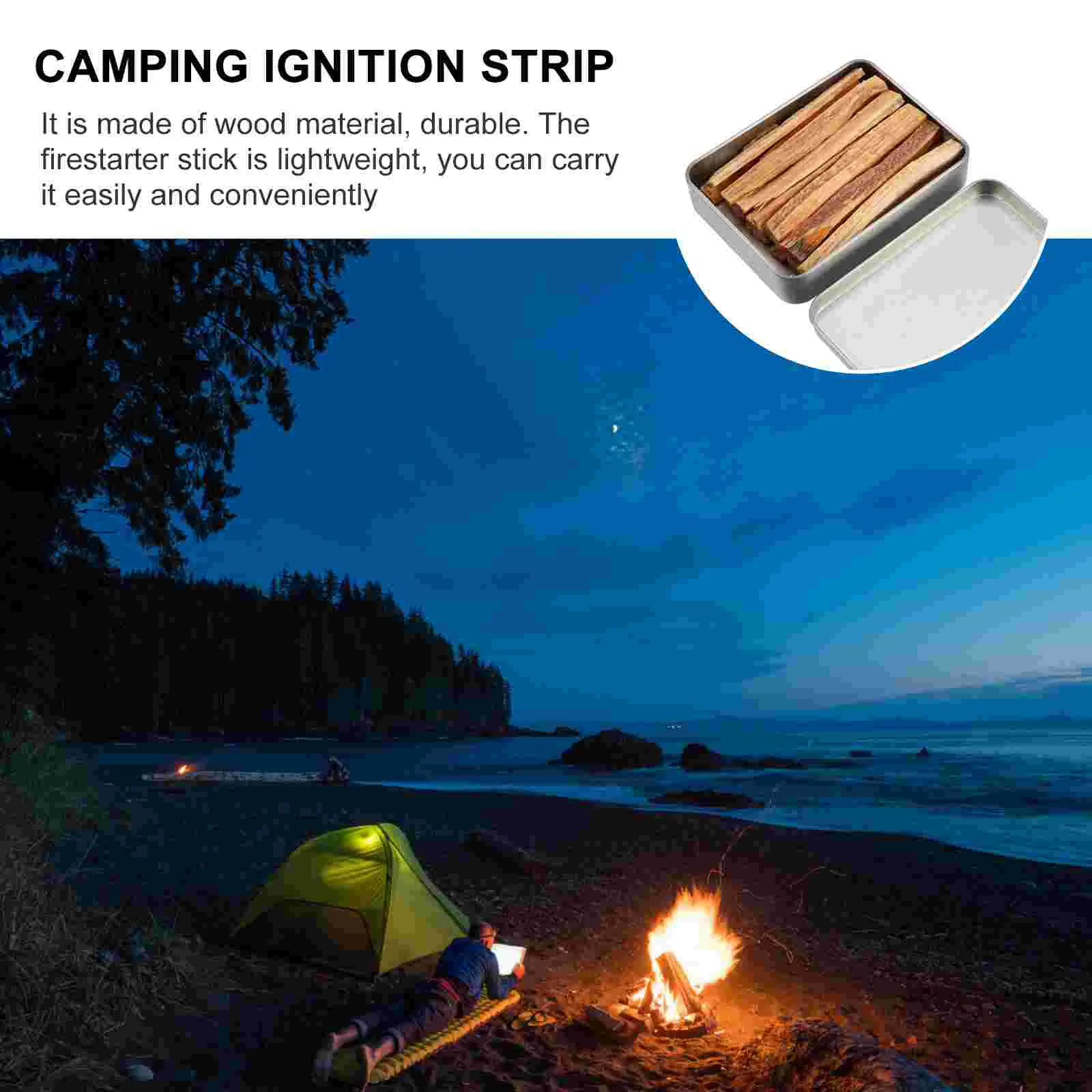In this image, a camper is spending dusk on a rocky beach next to the ocean. The sky is a darkening blue, signaling the approach of night. The beach features a green tent on the left and a large, roaring campfire on the right. The camper lies stomach-down on a sleeping bag or mat, absorbed in reading a piece of paper or possibly a tablet. In the distance, another small fire can be seen further down the beach near a jetty of pine trees extending into the water. Above the image, a white border contains bold, capitalized text that reads "CAMPING IGNITION STRIP," followed by a smaller black text detailing that the fire starter stick is "made of wood material, durable, lightweight, and can be carried easily and conveniently." To the side, an inset image depicts a rectangular silver tin filled with neatly stacked wood strips.